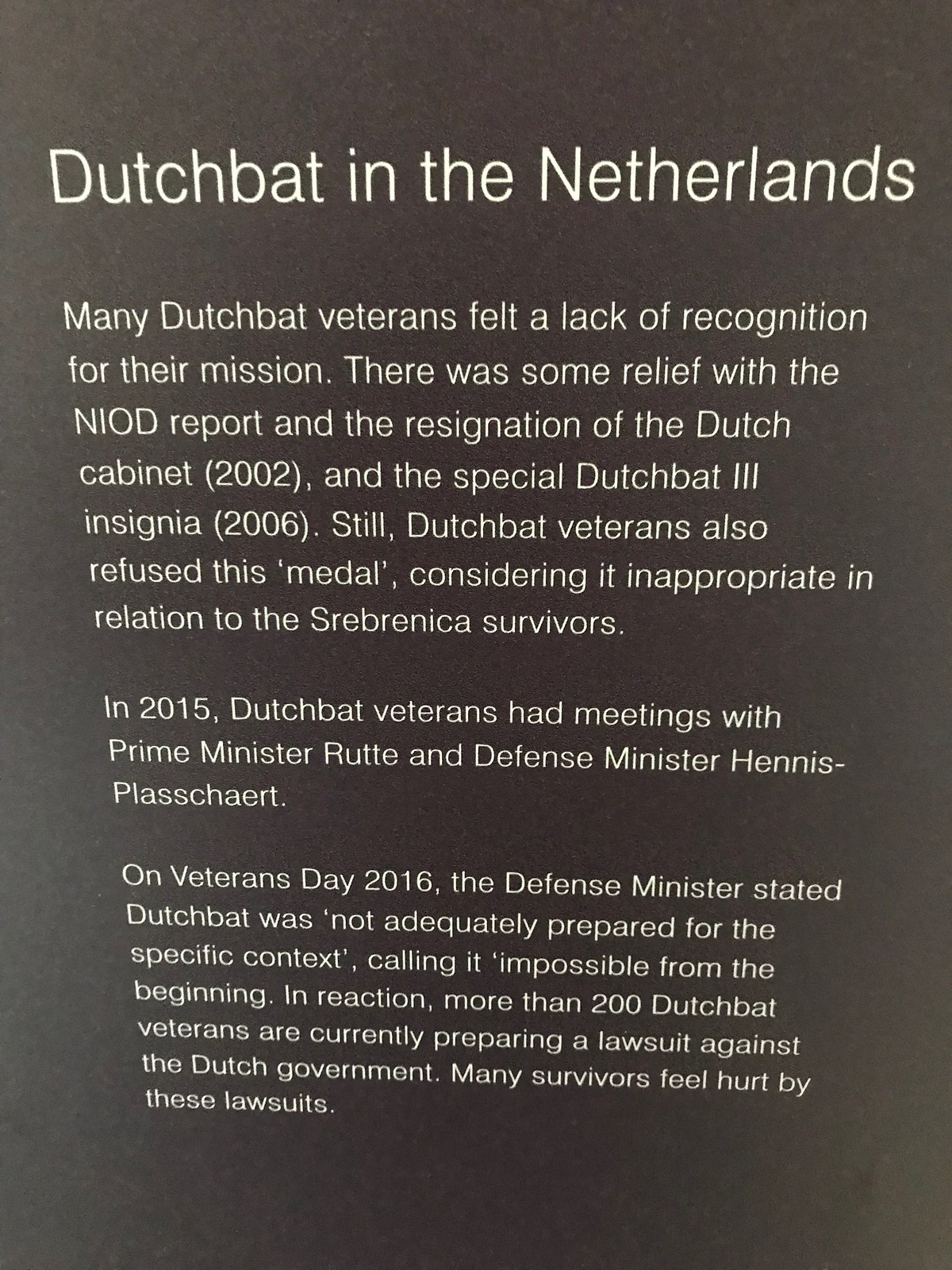An image featuring a black background with white writing is presented, detailing the experiences of Dutchbat veterans from the Netherlands. The words appear to be slanted, with the top text closer and the bottom text further away. The title "Dutchbat in the Netherlands" heads the image, followed by several paragraphs. The text explains that many Dutchbat veterans felt a lack of recognition for their mission, finding some relief with the NIOD report and the resignation of the Dutch cabinet in 2002, as well as the introduction of the special Dutchbat III insignia in 2006. However, the veterans refused the medal, viewing it as inappropriate in relation to Srebrenica survivors. In 2015, Dutchbat veterans met with Prime Minister Rutte and Defense Minister Hennis-Plasschaert. On Veterans Day 2016, the Defense Minister acknowledged that Dutchbat was not adequately prepared for their specific mission, deeming it impossible from the beginning. In reaction, over 200 Dutchbat veterans are currently preparing a lawsuit against the Dutch government, causing hurt among many survivors.